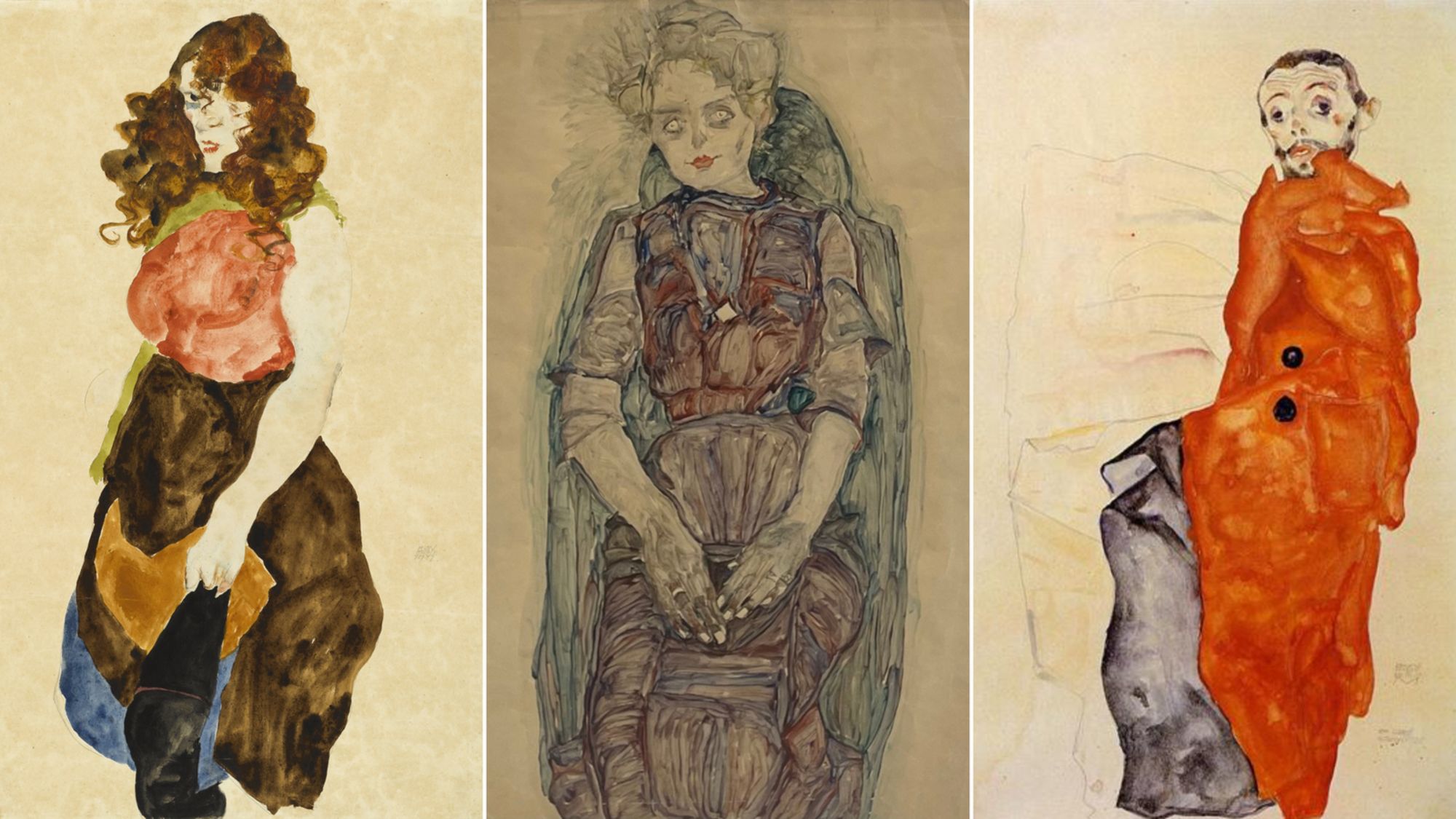The illustration features three distinct yet peculiar portraits of people rendered in a mix of sketch and colorful styles. The first portrait depicts a mysterious woman with curly brown hair partially obscuring one of her eyes. She dons an orange top and a skirt with varied hues of brown, yellow, and blue, revealing black pants underneath. The second portrait showcases a woman with short blond hair, yellow eyes void of pupils, lending her a possessed appearance. She's dressed in older-style formal clothing, sitting in a gray chair with her hands resting on her lap. The final portrait portrays a man shrouded in an orange coat with two black buttons, giving a vampiric and unsettling vibe as his arms and legs seem indistinct under the coat, which drapes over black trousers, enhancing his eerie appearance.